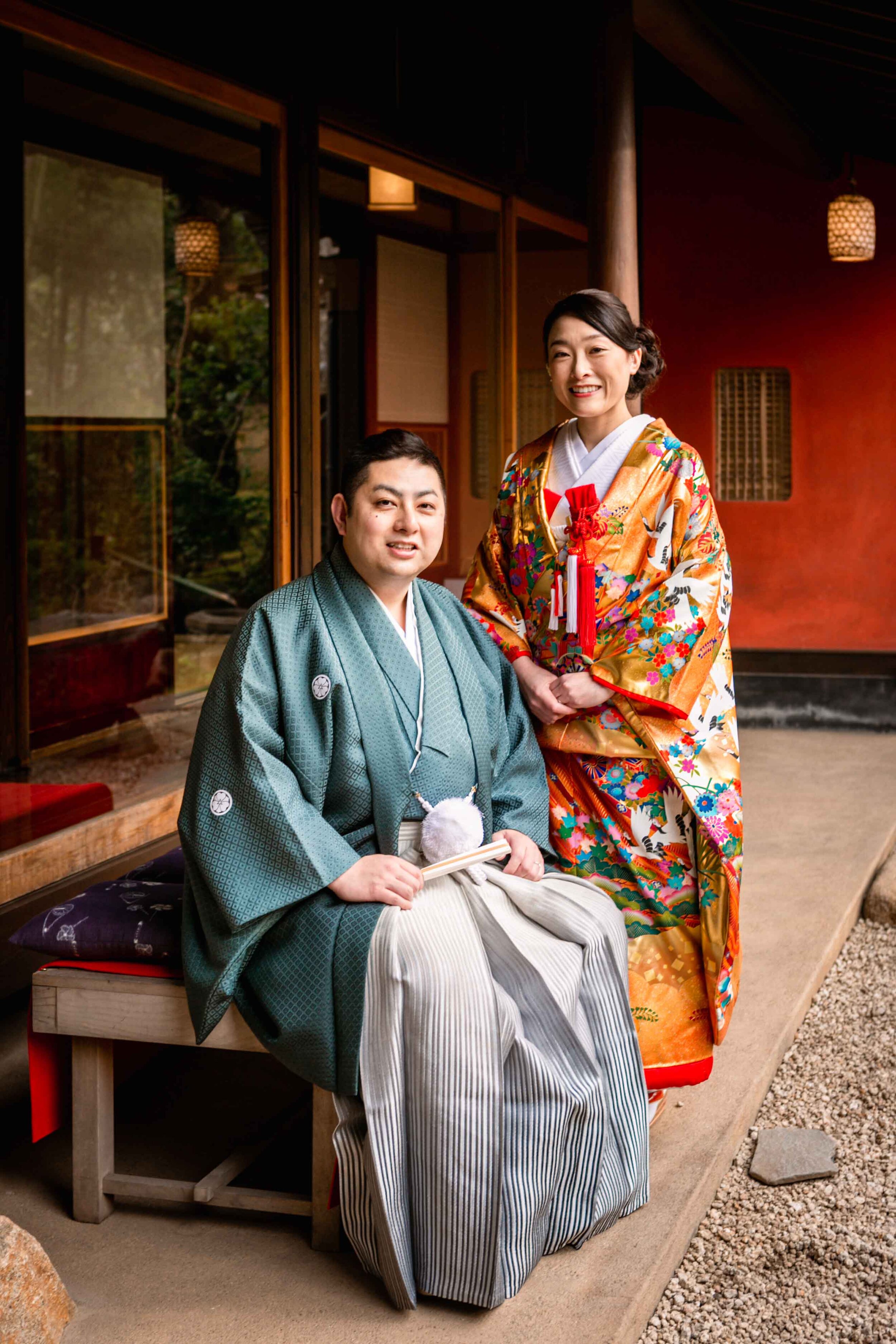This high-resolution color photo depicts an Asian couple, likely of Japanese descent, in traditional pre-Western Japanese attire. The man, who has short brown hair, brown eyes, and a slight smile, sits on a wooden bench. He wears a jade green robe with black and white vertical stripes on the lower part covering his legs, and he holds a fan. The woman stands beside him, her brown hair styled in a bun. She is dressed in a vibrant kimono with an orange base adorned with colorful flowers and birds, and her inner clothing is white. A red necklace adorns her neck, and she smiles gently. The couple is situated in front of an orange building with Japanese tea lanterns and three windows reflecting nature. The scene sits atop a concrete pavilion with gravel visible in the bottom right corner, indicating they are in a Japanese garden setting.